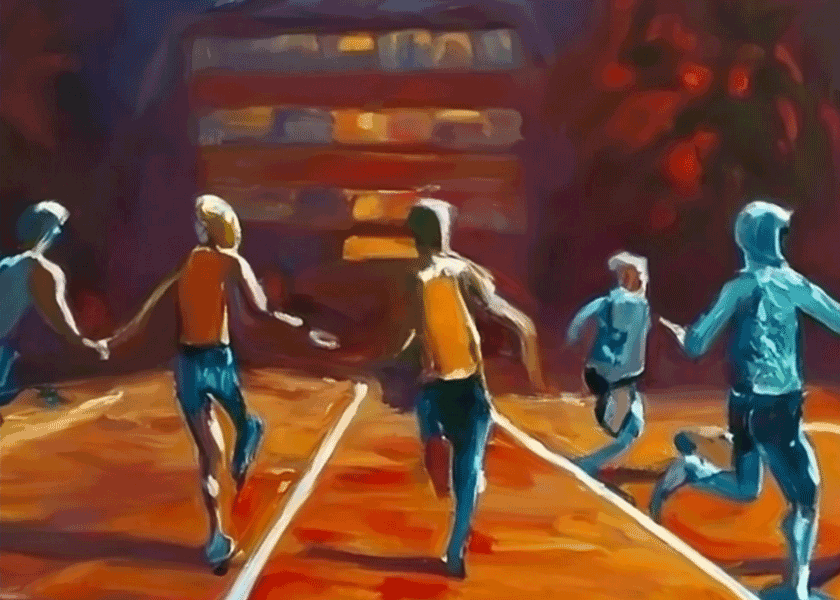The image is a detailed and vibrant mural depicting a race scene with a warm and intense color palette dominated by orange, red, and scattered blue elements. The ground of the mural features reddish-orange tracks with white lines demarcating separate lanes. In the center three individuals are linked hand-in-hand, suggesting they are in a relay race. The leftmost figure wears a blue t-shirt and has extended his right arm to hold the left hand of the next person, who is dressed in an orange-red tank top and blue jeans; this middle person appears to have blonde hair. The middle runner extends his right hand to the third participant, who is wearing a yellow shirt with blue jeans and appears to be leading the group. 

In the background, to the top right, there is a faint outline of a multi-story building with lights on, and possibly indistinct features like clouds or mountains, adding a layer of depth. Two more figures can be seen towards the far right side of the mural; one in blue seems to be moving off to the side or towards another person who might be preparing to join the race. The overall scene is dynamic yet somewhat surreal, with distorted figures and a blocked-off finish line, adding an element of mystery to their race's conclusion.